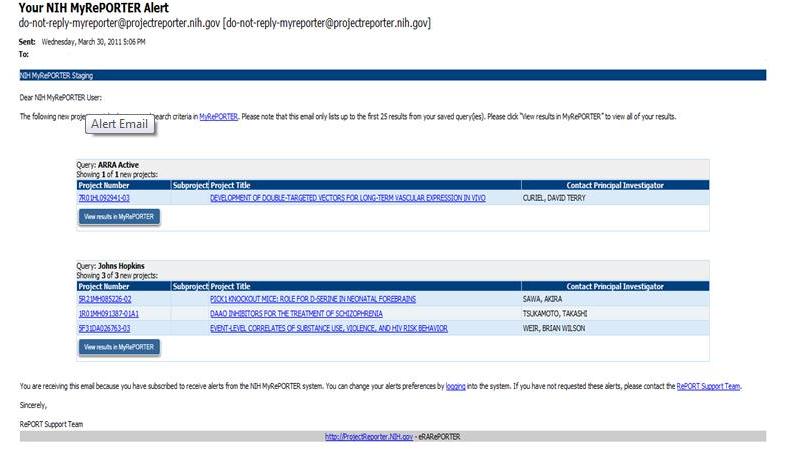This webpage displays an email notification from the NIH My Reporter system. The interface is predominantly white, featuring various sections of text. At the very top, it reads "Your NIH My Reporter Alert," followed by an email address: donotreplymyreporter@projectreporter.nih.gov. The email was sent on Wednesday, March 30th, 2011, at 5:06 PM.

Below, a blue bar labeled "NIH My Reporter Staging" stands out. The text immediately under this bar begins with a greeting: "Dear NIH My Reporter User," and continues to inform the recipient about new project research criteria updates in My Reporter. It notes that the email includes only the first 25 results from saved queries and advises clicking "View Results in My Reporter" to see all results.

There is a box titled "Query ARRA Active," showing one new project with relevant details such as the project number, title, and a blue "View My Reports" button. Another section labeled "Query John Hopkins" indicates three new projects, each with their respective project numbers, titles, and the principal investigator's contact information.

At the bottom of the email, a notification explains that the recipient is receiving this alert because they subscribed to NIH My Reporter notifications and provides instructions for changing alert preferences by logging into the system. It also advises contacting the report support team if the alerts were not requested. The text is mainly in black, with numbers and clickable links highlighted in blue.